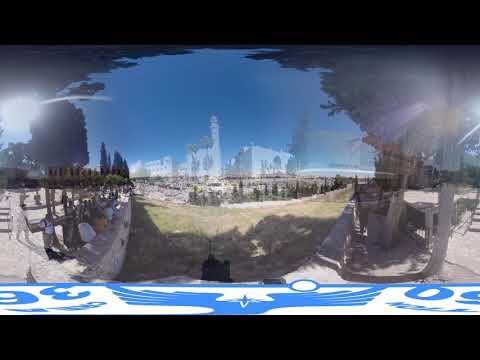This rectangular image, approximately three inches wide by two inches high, presents a complex and layered scene combining multiple visual elements. At its core, it displays a green grassy field centrally positioned, flanked by light stone-colored walls and alcoves on both the left and right sides. On the left, a raised stone platform with indistinct tourists, some carrying backpacks, overlooks the field. In the background, a distant white stone city is faintly visible, creating an impression of transparency suggestive of an ancient place, potentially reminiscent of a historical site like a sports arena in Greece.

Overlaying this central image is a partially transparent photograph of a modern cityscape, complete with tall buildings and a prominent white tower in the middle. This double exposure effect lends a warped and surreal quality to the scene, making it appear as if viewed through distorted Plexiglas.

Across the bottom of the image, beneath a black footer, a band with a white background and a blue stripe at the top contains a blue eagle logo. Accompanying this emblem are blue numbers, with ‘360’ prominently displayed, indicating a 360-degree view, albeit upside down in parts.

Overall, the image blends historical and modern elements with a reflection-like clarity, creating a puzzling yet captivating visual narrative.